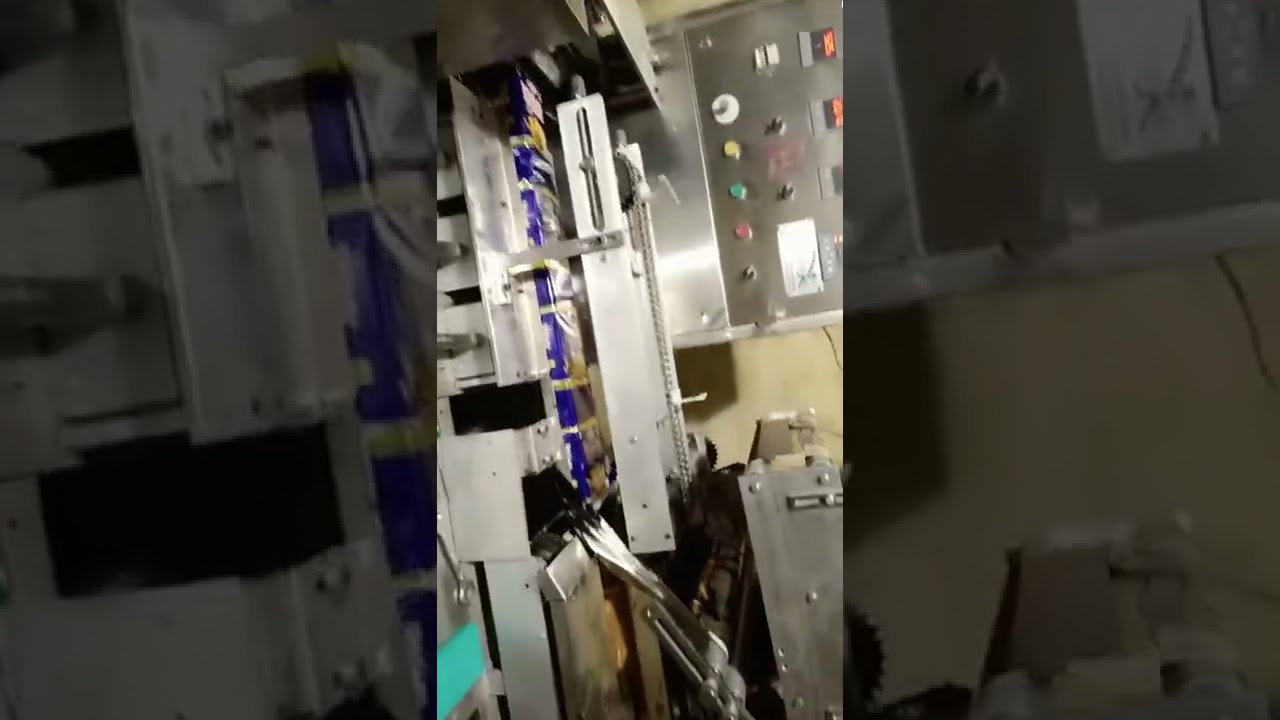The image depicts a cluttered room filled with intricate machinery, primarily composed of angular, shiny silver metal with various rivets and connections. The equipment features buttons and dials of diverse colors, including red, yellow, green, white, and black, along with silver knobs. Prominent in the upper right corner, a section of metal cabinetry attached to the tan or light mustard-colored wall houses an array of buttons and toggle switches. Notably, the machinery is organized into three distinct layers, with some parts appearing to descend inward. Blue items and packages are scattered among the machinery, adding splashes of color. The image is vertically oriented, making it more challenging to discern the overall context or function of the machinery, possibly located within a factory setting. The left and right sides of the image feature a wide, dark border, showcasing blown-up, faded-out elements from the main picture for emphasis.